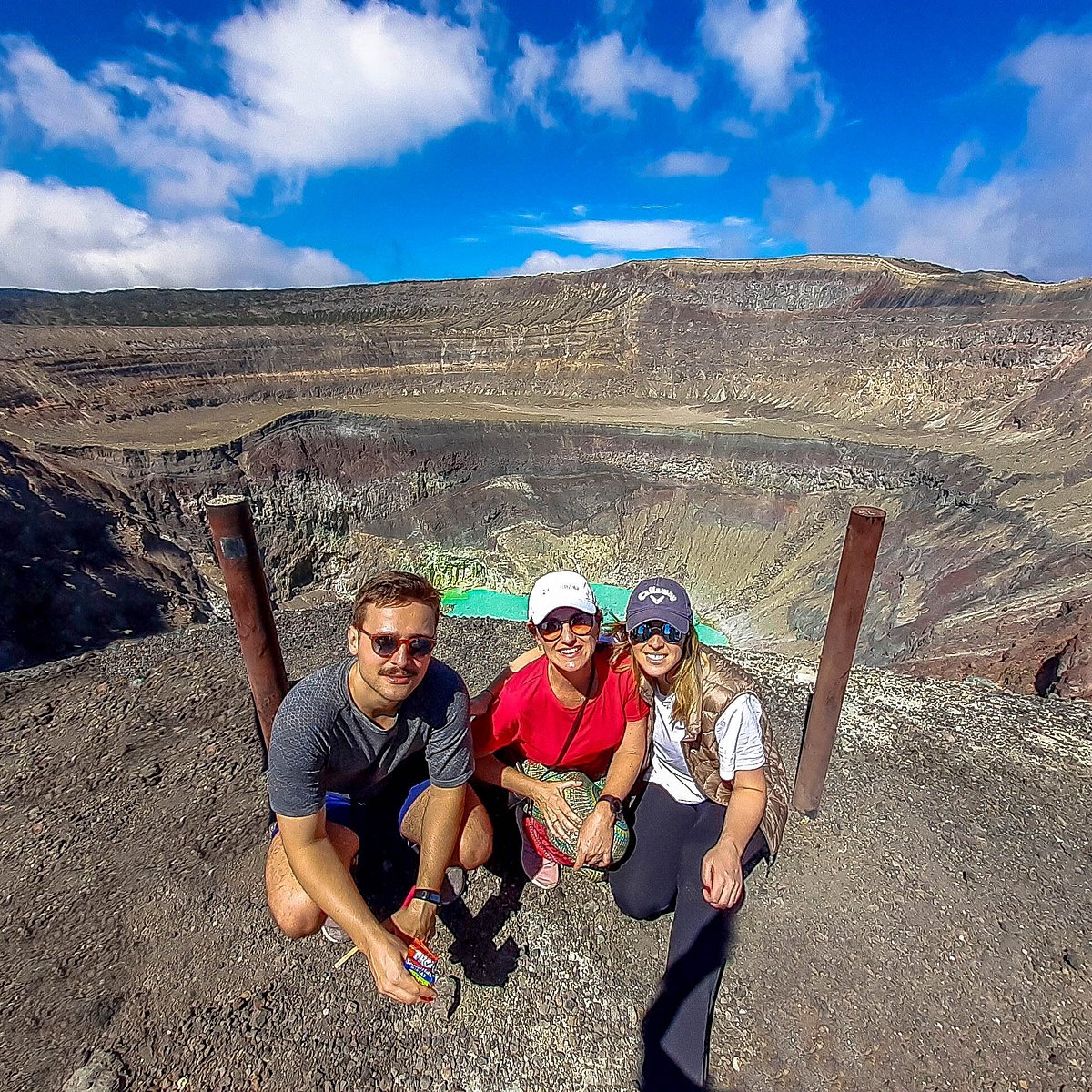This vibrant outdoor photograph captures a group of three Caucasian friends smiling and kneeling on the edge of a dramatic cliff that descends into a vast crater, possibly reminiscent of the Grand Canyon. The central figures are dressed for a hike, exuding a sense of adventure and camaraderie. 

The man on the left wears sunglasses, a gray t-shirt, and blue shorts, with a prominent brown mustache and short brown hair. Flanked in the middle, a woman with a white baseball cap and sunglasses dons a red shirt and green print leggings or pants. Her crouched posture mirrors that of the man beside her. To the right, another woman has her arm around the central woman, sporting a darker baseball cap, sunglasses, and a combination of a brown vest, a white t-shirt, and black pants. 

The dynamic scenery showcases further ridges ascending from the crater in the background, under a bright blue sky adorned with puffy white clouds. Enhancing the scenic beauty, a small pool of aqua-blue water lies at the bottom of the crater, while two brown fence posts frame the friends on either side, creating a balanced composition that amplifies the grandeur of their surroundings.